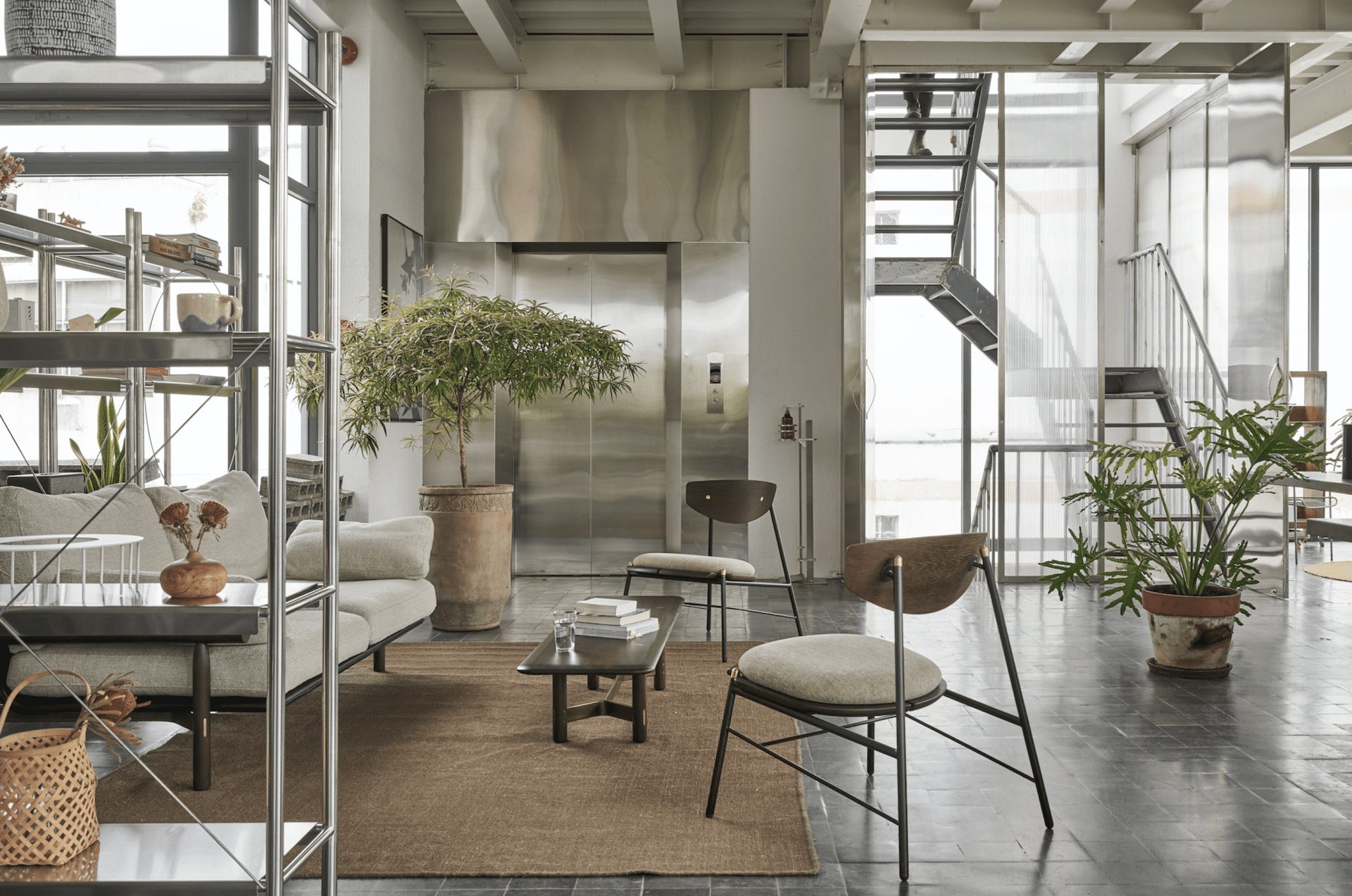This detailed and vibrant horizontal rectangular photograph showcases the interior of a highly modern home, filled with sleek and metallic design elements. The open and airy room is bathed in natural light streaming through the large windows that punctuate the space. Dominating the central area is a stylish couch with wooden legs, complemented by two hyper-modern metal chairs. A wooden coffee table, adorned with books and a glass with ice, stands on a brown floor rug. To the left, a metallic shelving unit is stocked with various items, and a couch alongside a potted plant enhances the modern aesthetic. 

In the background, an elevator is visible, indicating a touch of luxury. A striking open metal staircase with landings ascends to an upper level, and a person's legs are seen mid-climb. The room also features multiple plants, including a large tree in a traditional planter and another sizable plant on the right in a decorative pot. Concrete blocks appear near one of the many windows, adding to the room's contemporary vibe. The clarity of the image, combined with the abundance of natural light, emphasizes the clean lines and modern features of the setting, making it a perfect example of hyper-modern interior design.